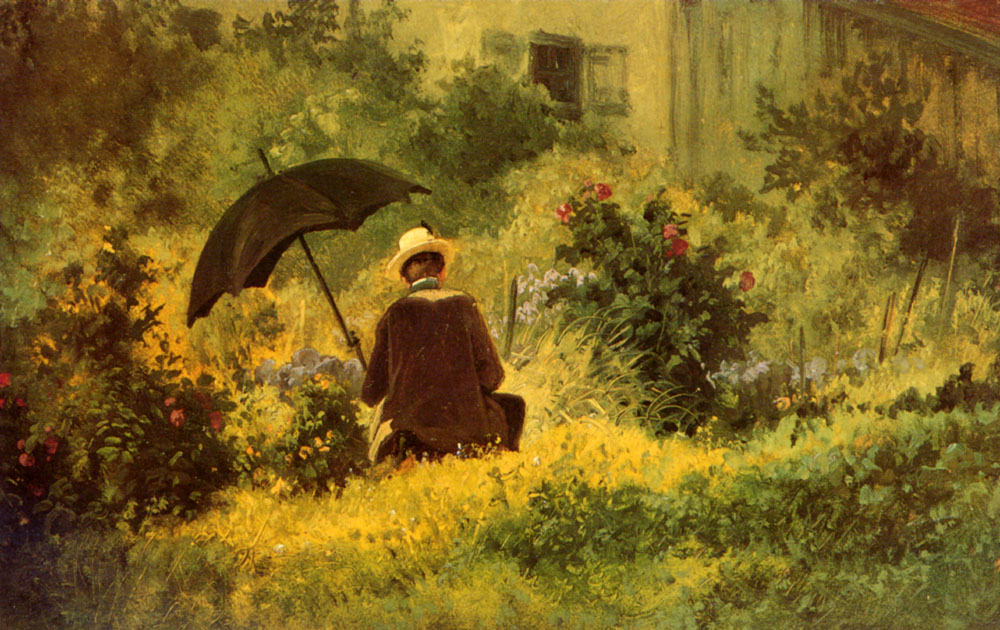In this detailed oil painting, a man sits alone amidst a lush, vibrant garden, captured in an exquisite blend of colors and textures. His back is turned to the viewer, revealing his brown hair beneath a tan hat. He wears a dark brown jacket and brown pants, complemented by a green scarf. The man is positioned slightly off-center to the left, seated on the green grass, with a large black umbrella providing shade beside him. 

Surrounding the man are various bushes and colorful flowers, including vibrant red roses and an array of yellow, blue, and white blossoms. The greenery is rich and varied, with light and dark green hues interspersed among the trees and bushes. To his left, the dense foliage is punctuated by flashes of color from the diverse plant life.

In the distant background, partially obscured by the lush garden, stands a house painted in a greenish-yellow hue. A brown window is visible, giving a glimpse into the home's exterior, which further suggests the setting could be a backyard. Trees with dark green leaves reach above him, framing the scene and adding depth to the composition. This idyllic, serene environment is lovingly rendered with the skillful brushstrokes characteristic of classic oil painting.